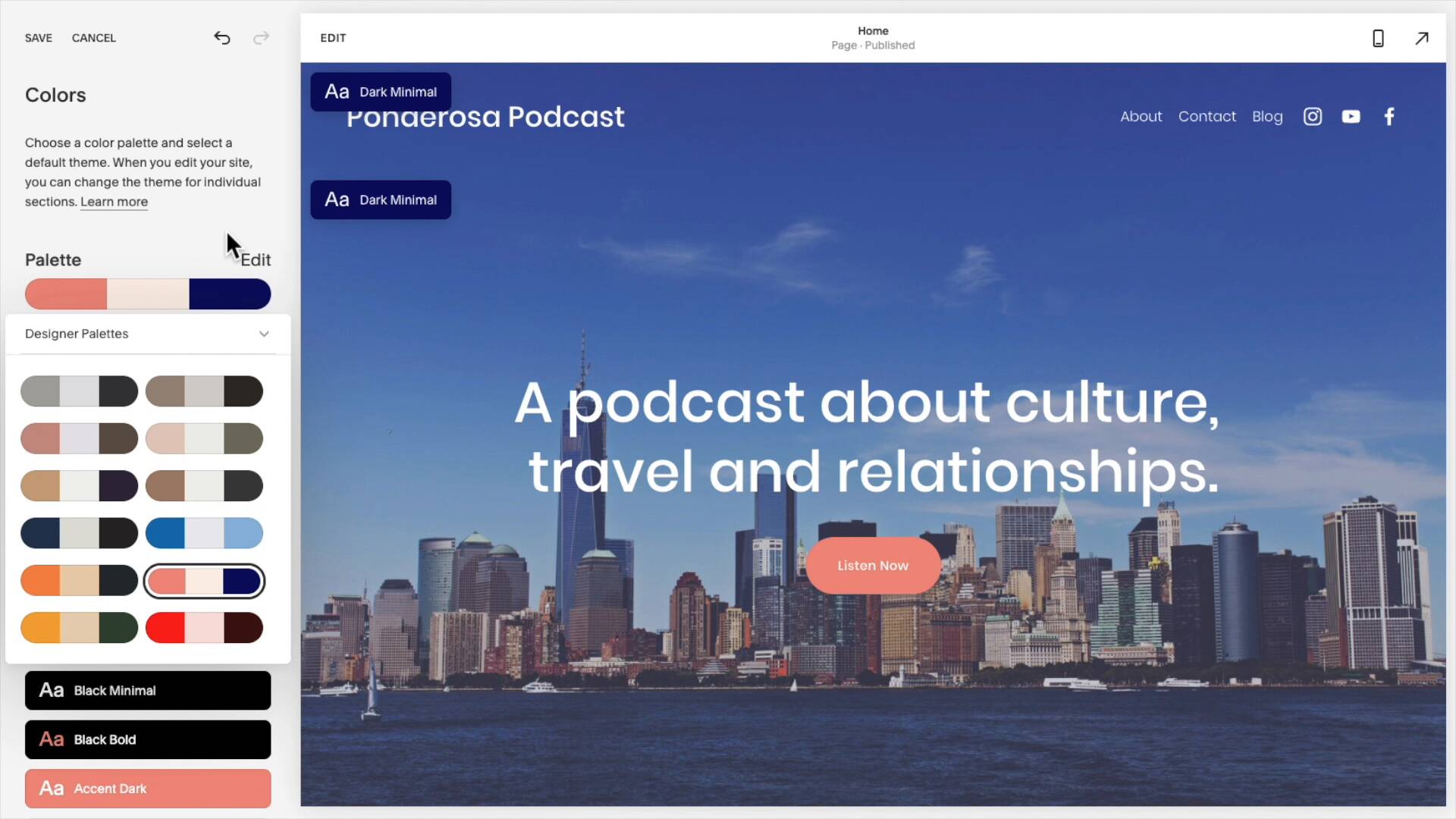This is a detailed screenshot of a web page design interface, specifically showcasing the central part of the page. On the left side of the screenshot, there is a vertical gray panel featuring two buttons at the top left corner: "Save" and "Cancel." To the right of this panel, there are two navigation arrows; the arrow pointing to the left is dark gray, while the arrow pointing to the right is light gray.

Beneath these arrows is a section labeled "Colors." The word "Colors" is displayed in a bold black font. Directly below this heading, there is a description, followed by labels "Palette" on the left and "Edit" on the right. In the following section, there is a bubble showcasing three distinct color swatches: dark pink, light pink, and blue. Below this bubble, there is a panel where you can change the palette, and the selected palette is encircled in blue.

Further down, the interface lists additional categories: "Basic Minimal Font," "Black Bold Font," and "Accent Dark." The "Accent Dark" category is selected and marked with a pink box for emphasis. At the top right corner of the page, there is a “Home” button. The main body of the page features a large image with a text overlay, providing a visual representation of the design being edited.